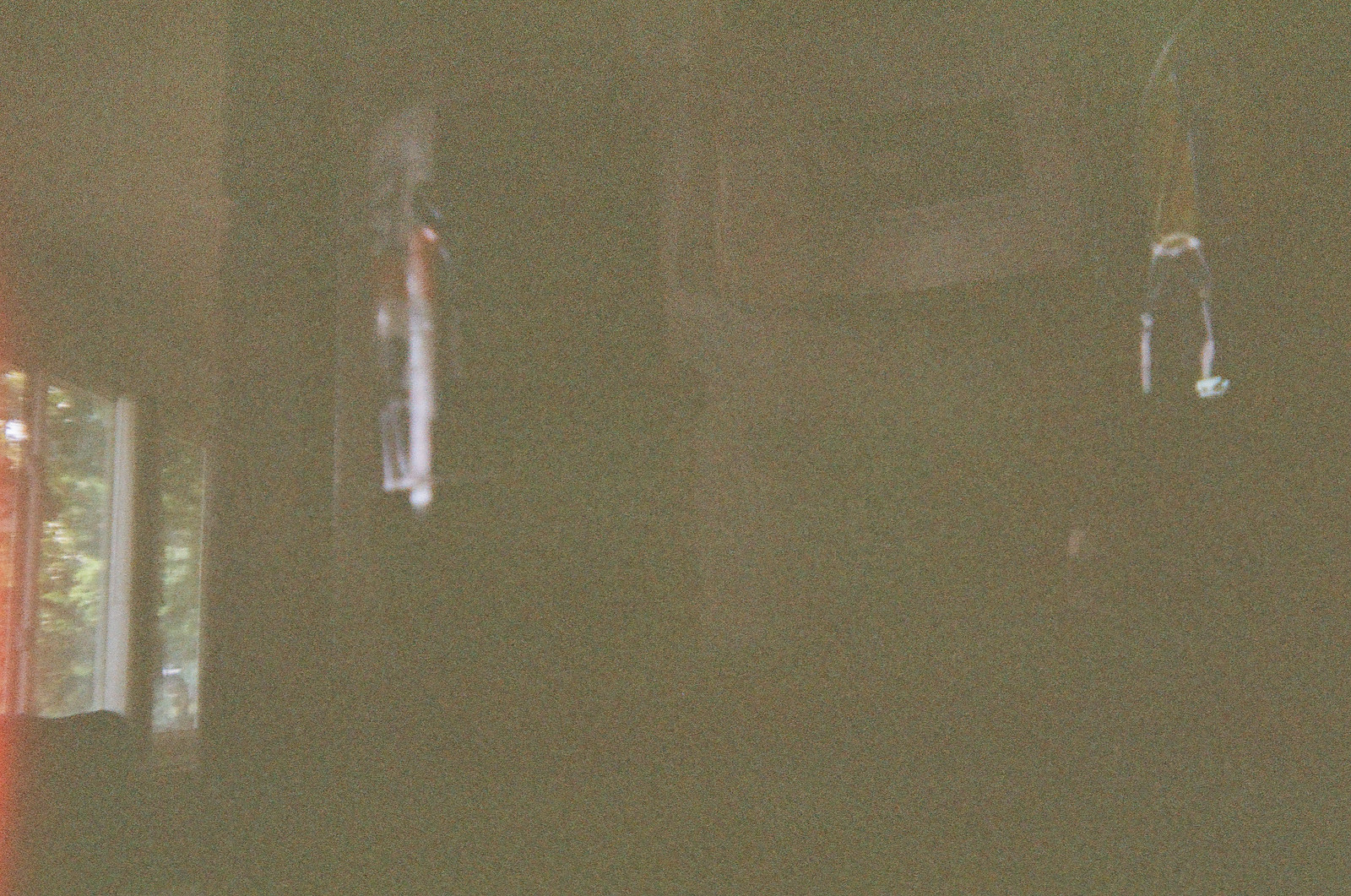This photograph, taken indoors under poor lighting conditions, is both blurry and grainy, plagued with significant visual noise. The upper part of the image features a light-colored rectangle with a darker inset, likely a thermostat with a digital display mounted on a wall. Adjacent to this is an irregular bronze and white shape. Towards the left side, a vertical white line is visible with an orange form near its top, and to the extreme left edge, a window reveals the faint outline of trees outside. Despite the window allowing some light into the room, it remains dim, casting ambiguity over the scene. Two metallic objects can be seen hanging from the ceiling, one on each side of the image. Between them, a silver microwave with a black rectangle is discernible, possibly situated above a stove, though the stove is indeterminable. Additionally, a shirt or similar item appears to be hanging to dry, adding to the room's cluttered and enigmatic appearance. The room's overall dimness and the photograph's poor quality render the details exceedingly difficult to distinguish.